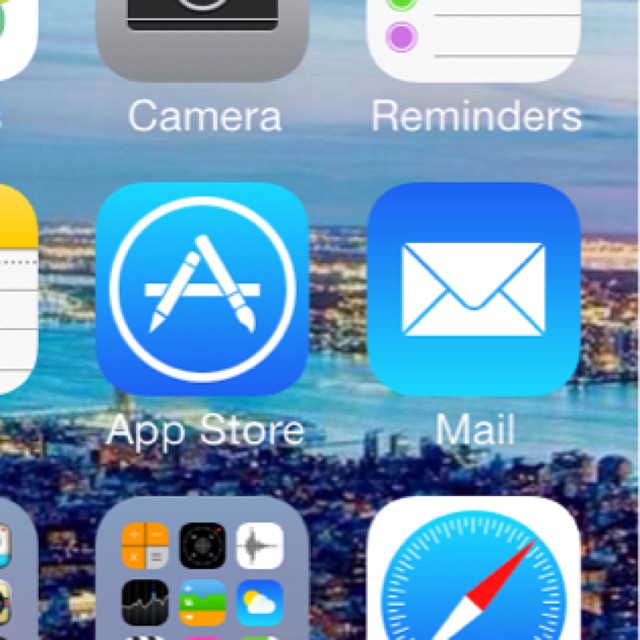**Detailed Caption:**

This image is a screenshot of a camera interface displaying a cityscape background. The vibrant city image showcases numerous illuminated buildings and lights, with a prominent river flowing through its center. Above this lively urban scenery, a light blue sky dotted with scattered clouds completes the backdrop.

At the top left corner of the screen, a partial white icon is visible, though its exact nature is indiscernible. Adjacent to it is a classic gray icon box featuring the bottom of a black camera icon, with the label "Camera" written in white text underneath.

To the right of the camera icon is the white reminders icon, which resembles a notepad with a small purple circle and a line. Below this, the word "Reminders" is written in white text.

In the row below, starting from the left, there is a partially visible notepad icon. The top portion of this icon is yellow, transitioning into a white section with lines. Next to it is the App Store icon, characterized by a blue background and a white circle enclosing a paintbrush and a pencil. The text "App Store" appears beneath this icon.

Adjacent to the App Store icon is the classic mail icon, which consists of a blue rounded square with a white envelope in the center, accompanied by the label "Mail" beneath it.

Proceeding to the row below, from left to right, there is a folder containing multiple icons, although the exact icons are not distinguishable. To its right is another folder that contains various application icons, such as the Compass, Weather, and Calculator apps, a total of six icons arranged in two rows of three.

Lastly, the Safari icon is positioned next to this second folder. It is depicted as a white rounded square with a blue center, featuring a compass design. The compass displays a red directional arrow pointing to the upper right, and a white arrowhead at the bottom.